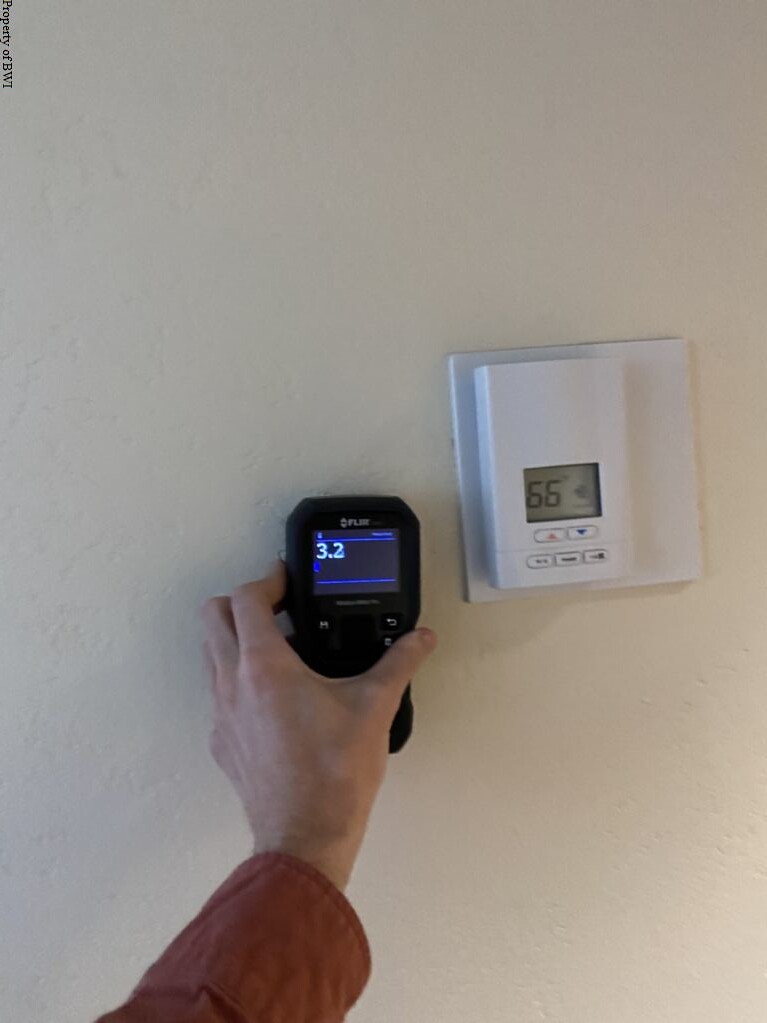In this image, the viewer's focus is drawn to several key elements against a plain white wall backdrop. In the very top left corner, the phrase "Property of BWI" is prominently displayed in black lettering, though it’s partially cropped by the edge of the photo. The lower portion of the picture features a hand, cut off just at the wrist, emerging from the bottom edge. The hand is dressed in a long-sleeve shirt of a vibrant orange color and is holding a black stud finder. The stud finder is marked with the number "3.2" in white, flanked by blue lines above and below the number. The device itself has three buttons, the most visible of which has a circular arrow pointing left.

Adjacent to the stud finder, a thermostat is mounted on the white wall. The small rectangular thermostat is encased in a slightly larger white square and displays a temperature of "66 degrees." It includes five buttons: two at the top, adorned with indistinct red and blue symbols, and three at the bottom, which bear unclear black icons or lettering.